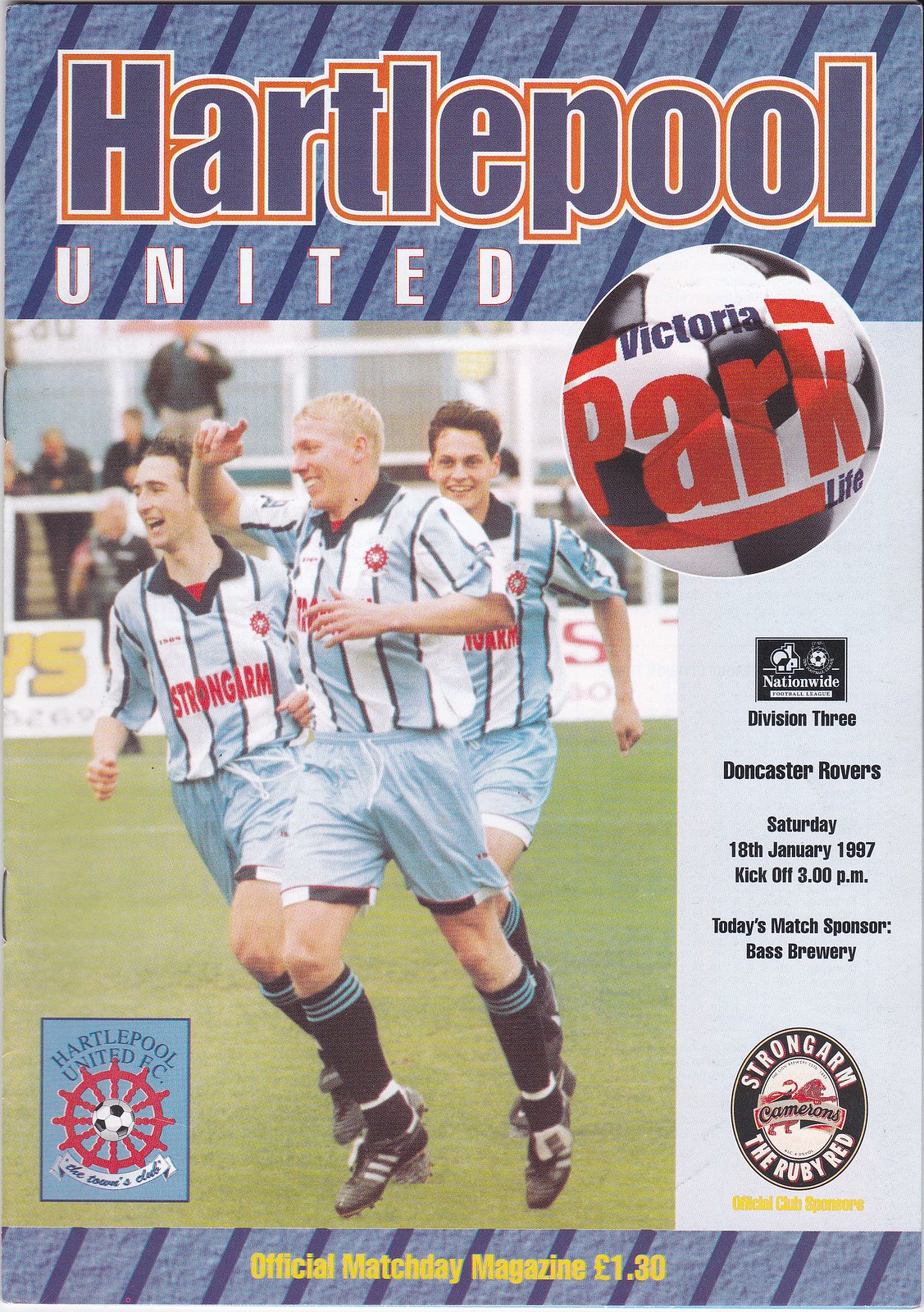This is the front cover of a football (soccer) magazine for Hartlepool United, featuring detailed design elements and information for an official match day. At the top center, "Hartlepool United" is prominently displayed in navy blue text bordered by white and orange. Below this, a graphic of a soccer ball contains the text "Victoria Park Life." Central to the image are three young players jumping in the air, dressed in cleats, black socks, light blue shorts, and striped white and light blue polo shirts. The shirts have a red logo that likely says "Strongarm." To the right of the players, details of the match are listed: "Division 3, Doncaster Rovers, Saturday, 18th January 1997, kickoff 3 p.m." Additionally, the match is sponsored by "Bass Brewery," featuring their "Strongarm" ruby red ale. At the bottom, in bold yellow font, "Official Match Day Magazine" is stated, along with the price "£1.30."